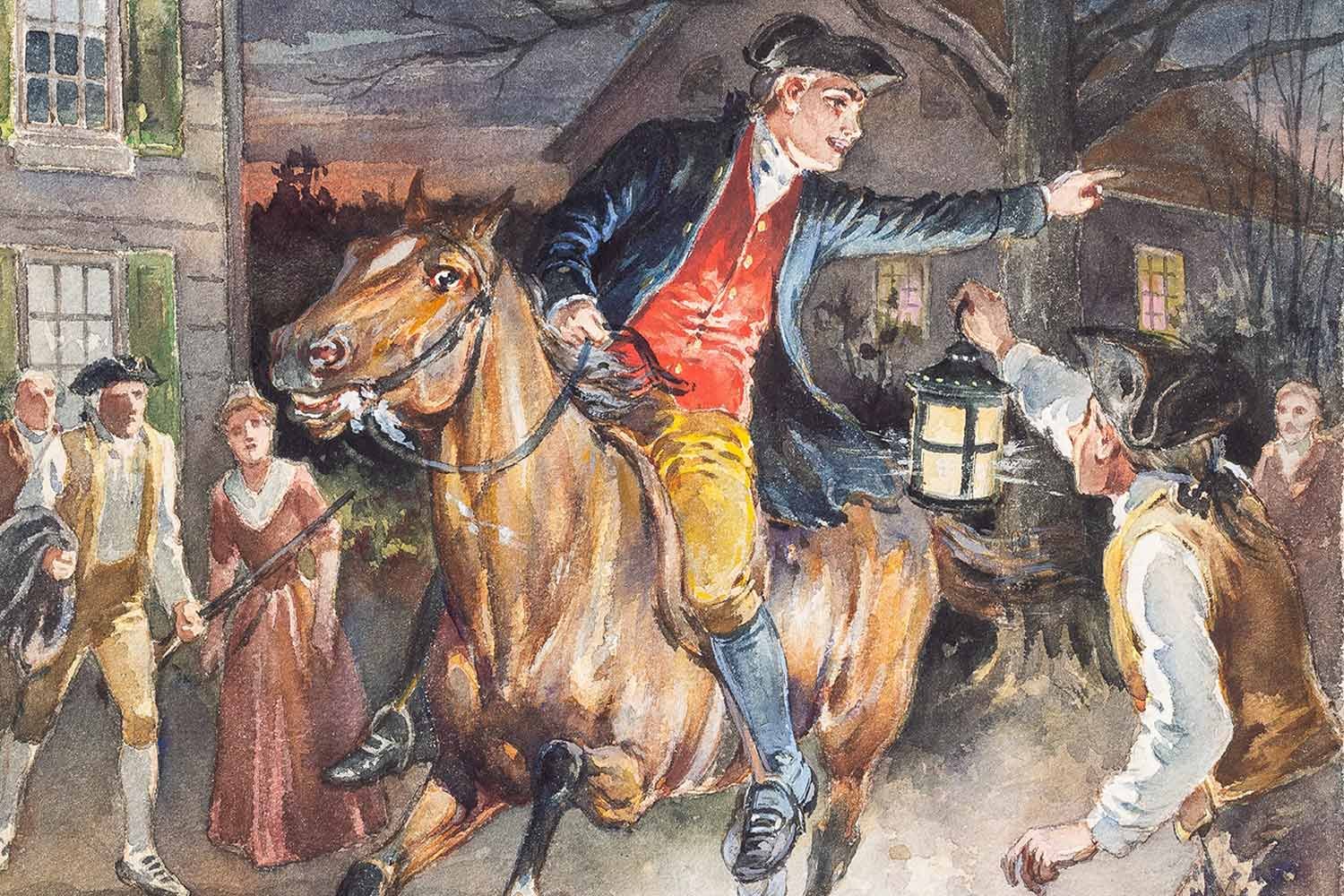The painting vividly depicts the midnight ride of Paul Revere. Set against the backdrop of a dusky evening, Revere is seen in full colonial attire—an eye-catching red vest beneath a dark blue jacket, yellow riding shorts, and shoes with gold buckles—astride a galloping brown horse. His left arm extended behind him, he appears to be alerting the townsfolk, possibly shouting, "The British are coming, the British are coming!" 

The urgency of his mission is evident in his posture and the horse's full gallop, signaling that he is not stopping. Flanking him is a man holding a lit lantern, clad in a brown vest and colonial hat, seemingly engaged in urgent communication with Revere. In the foreground, a vigilant man has stepped out of his house armed with a musket, ready to spring into action, his coat thrown on hastily. 

On the other side of the horse, a woman in a long pink dress stands with another man, who is also armed. The scene is framed by colonial-style houses with green windows and lit lanterns, emphasizing the community's readiness and attention. The presence of trees and the glow of lanterns heighten the dramatic atmosphere of this pivotal moment in American history.